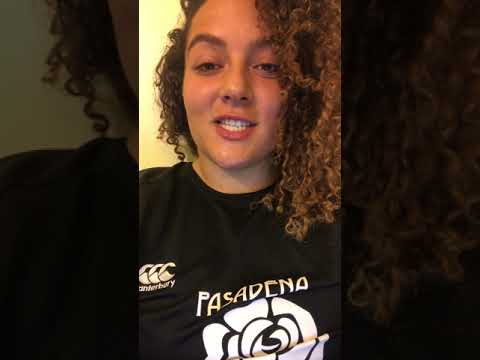The image depicts a young woman in her early 20s, potentially of mixed ethnicity, engaged in a video chat. She has tanned skin and curly, tight auburn hair. Her facial expression suggests she is in mid-conversation, with her mouth slightly open and her eyes appearing somewhat tired. She wears a black t-shirt featuring the word "Pasadena" written above a white floral design. Additionally, there is a logo on the left side of her chest, which includes three white circles and partially legible text resembling "A-N-T-E-R-B-U-R-Y." The background is a yellow wall, and the image has a unique effect where the sides are darker and magnified, particularly highlighting the left side of her face. The setting appears to be indoors, and the overall style suggests a still shot from a video blog or social media clip.